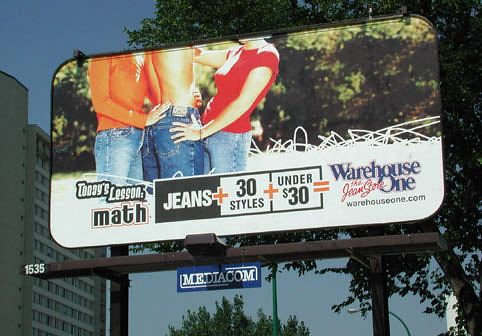This billboard advertisement features three individuals, positioned against a plain background. In the center stands a shirtless man, flanked on either side by two women, all of whom are clad in blue jeans. The woman on the left sports an orange long-sleeve shirt and has her hand playfully set just above the man's backside. On the right, the woman is dressed in a red short-sleeve shirt, gently resting her hand on the man's hip. The billboard text reads, "Today's Lesson: Math. Jeans + 30 styles + under $30. Warehouse One - The Jeans Store. WarehouseOne.com."